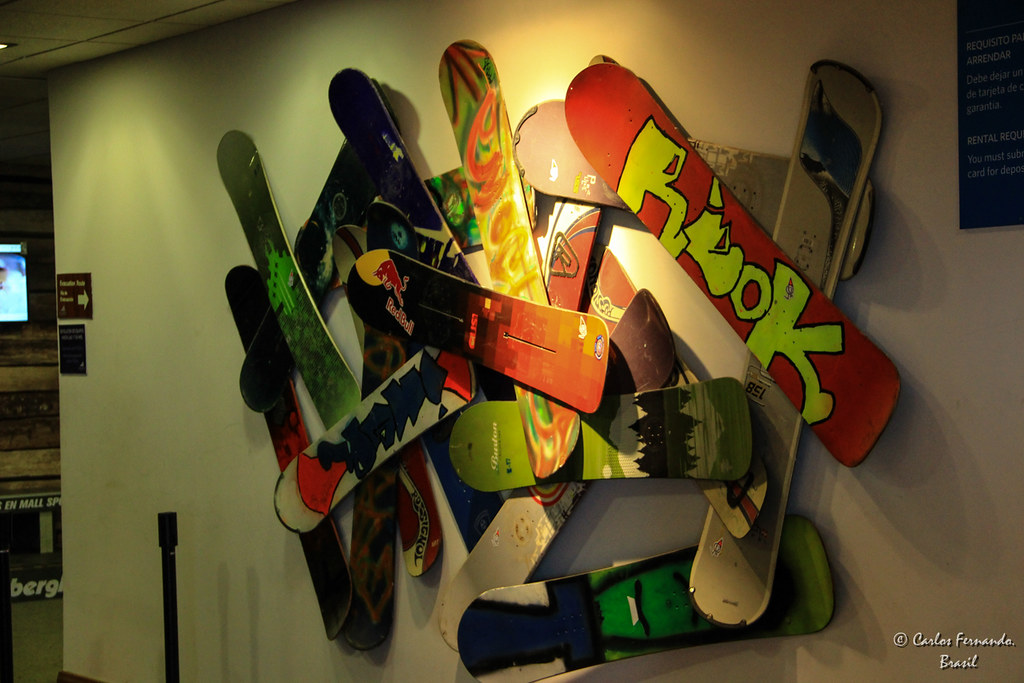This image depicts an art installation mounted on a wall, featuring roughly 12 to 15 colorful and overlapping skateboards that form a dynamic, almost chaotic arrangement. The wall behind this display appears to be a cream or beige color, with portions to the left in light green and to the right more distinctly beige, illuminated by spotlights that highlight the vivid artwork. The skateboards showcase a range of designs and colors, including red, yellow, green, white, light brown, and graffiti-style patterns. Notably, a red skateboard towards the top right has the letters "R-O-O-K" or "R-B-O-K" emblazoned in lime green. The installation appears to be in a public space, possibly a museum or gallery, as suggested by a black sign with a white arrow pointing right on the left side, indicating some form of navigation or direction. In the bottom right corner of the image, there's an inscription "Carlos Fernando, Brazil," in white font, attributing the artwork. A TV can be seen in the distance to the left, reinforcing the impression of a curated indoor setting.